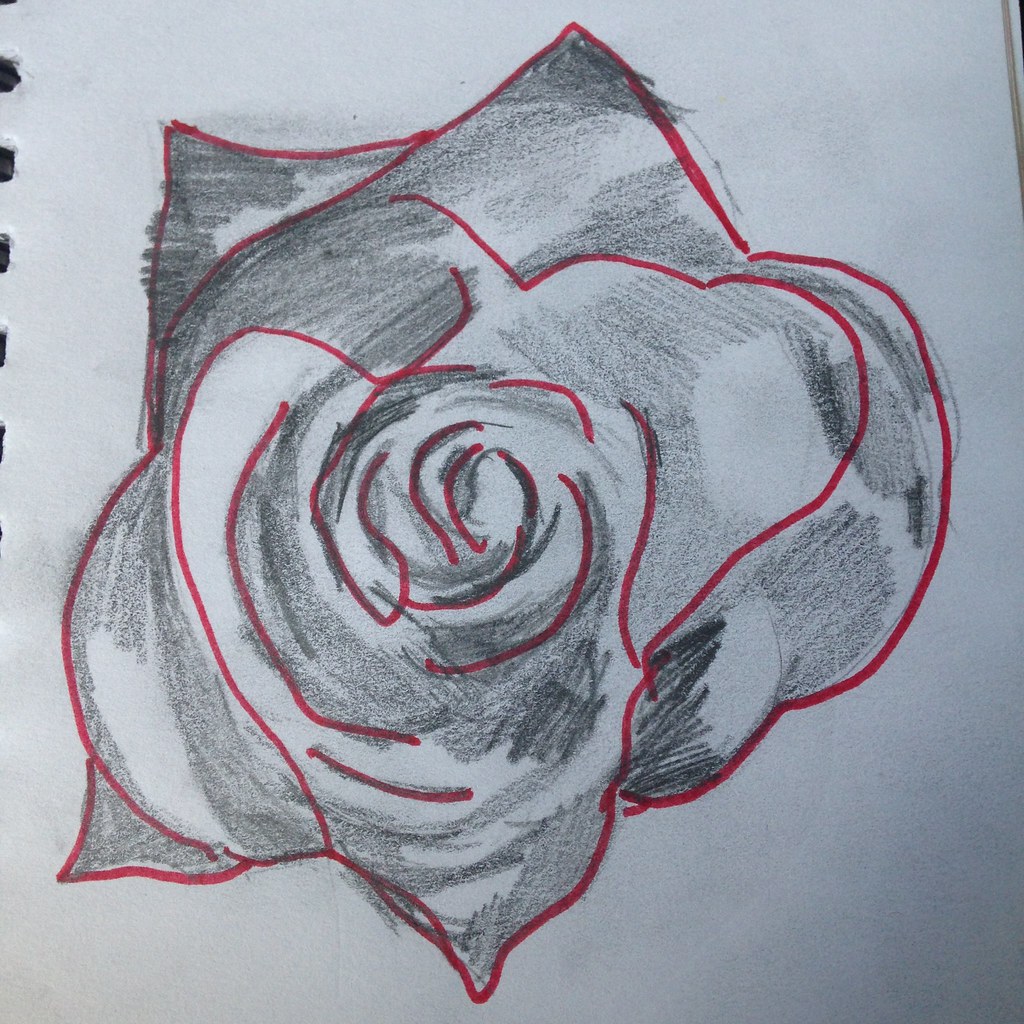This photograph depicts a sketch of a rose on a spiral-bound sketch pad. The left edge of the pad reveals a hint of its black, thick rings, indicating its spiral binding. The rose illustration is relatively simple, suggestive of an artist who may be new to sketching. The rose is identifiable by its design, with individual petals outlined in red marker. The outer petals are large and slightly pointed, while those closer to the center are smoother and more refined. The shading across the petals varies, with some areas showing darker tones and hints of highlights. However, the shading lacks cohesion, indicating a need for improvement in this technique.